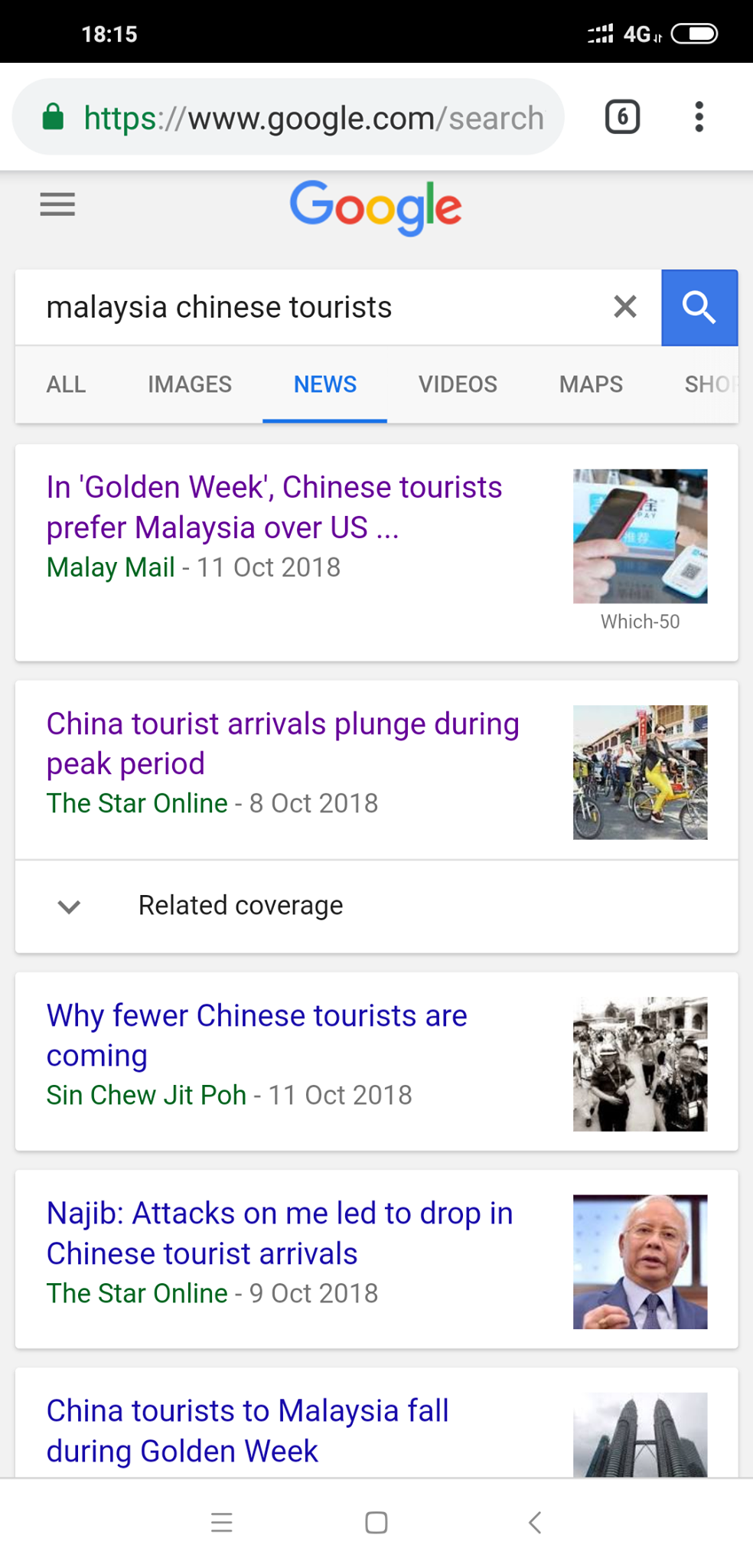The image features a Google search result page with a clean, light gray background. At the top left corner, there is a hamburger icon (three horizontal lines) indicating a menu. Below it, a prominently displayed search bar contains the phrase "Malaysia Chinese tourists" accompanied by an 'X' icon for clearing the search and a magnifying glass icon for search action.

Below the search bar, you can see various category tabs: All, Images, News, Videos, and Map. The main headlines are displayed in purple. The first headline is "During Golden Week, Chinese tourists prefer Malaysia over U.S." followed by the second headline, "China tourists arrivals plunge during the peak period."

Directly beneath these headlines is a section titled "Related Coverage" with a downwards arrow, indicating expandable content. The links under this section are in blue and include:
- "Why fewer Chinese tourists are coming"
- "Najib: Attacks on me led to drop in Chinese tourists arrivals"
- "China tourists to Malaysia fall during Golden Week"

On the right side of the screen, additional icons including a hamburger menu, a square, and an arrow pointing to the left are visible.